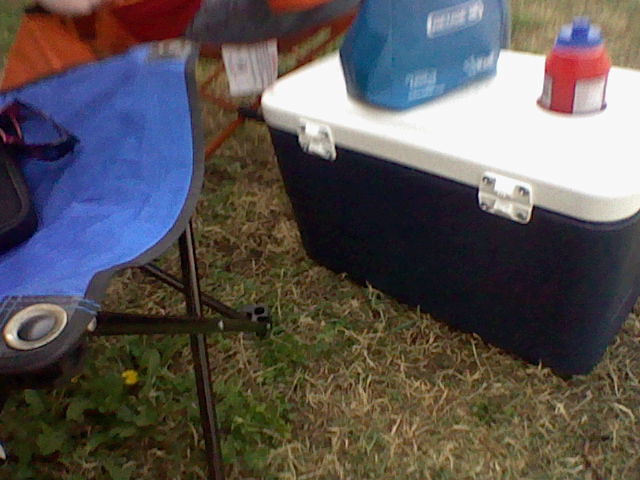This color photograph, though slightly blurry, captures a landscape orientation view of various camping gear set against a background of brown and beige grass with some vegetation. Central to the image is a large black cooler with a white hinged lid. The lid features a built-in space designed to hold a container. The cooler is set on the ground at an angle. On top of the cooler are a blue bag and a red can with a blue top. To the left of the cooler is a blue folding chair with drink holders, and to the right, there is a red (or possibly pink and orange) outdoor chair with a tag hanging off it. The entire scene exudes a sense of a casual outdoor excursion, with the cooler and chairs prepared for use on the dirt and grassy surface.